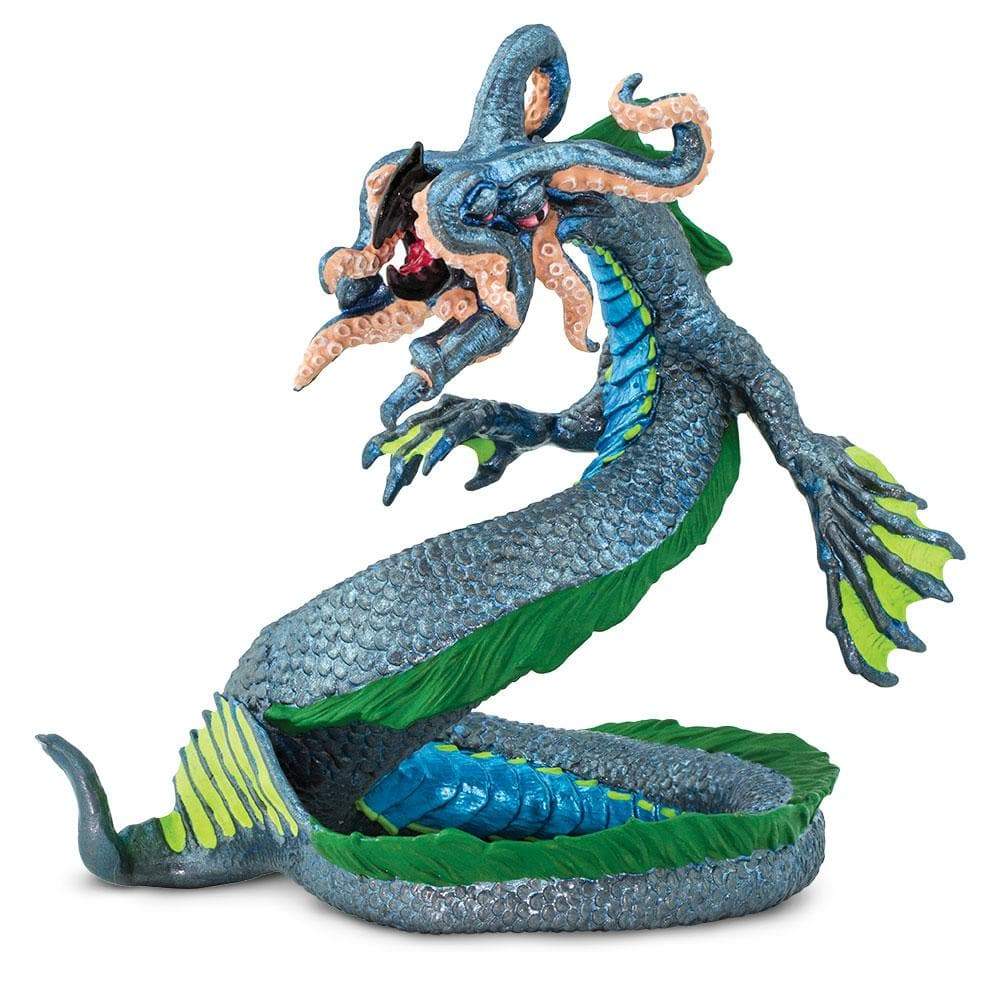The figurine depicts a grotesque and nightmarish monster, blending features of an eel, octopus, and dragon. Its long, slender body is covered in dark gray scales with a bluish undertone, accented by a green outline running down its back and light green spots peppering its tail. The tail also features blue lines and green outlines for added detail. The creature's head is a horrifying amalgamation resembling a squid, split down the middle with dual sets of eyes and a maw equipped with tentacle-like appendages. These tentacles mirror the grayish-blue scales and are lined with light pink suction cups. The monster has webbed, clawed hands with elongated fingers and green webbing between them. A prominent fin runs the entire length of its spine and tail, reinforcing its serpentine appearance. The figurine stands upright against a white background, emanating a sinister presence akin to a beast from a dark fantasy, perfectly suited for tabletop role-playing games like Dungeons and Dragons.